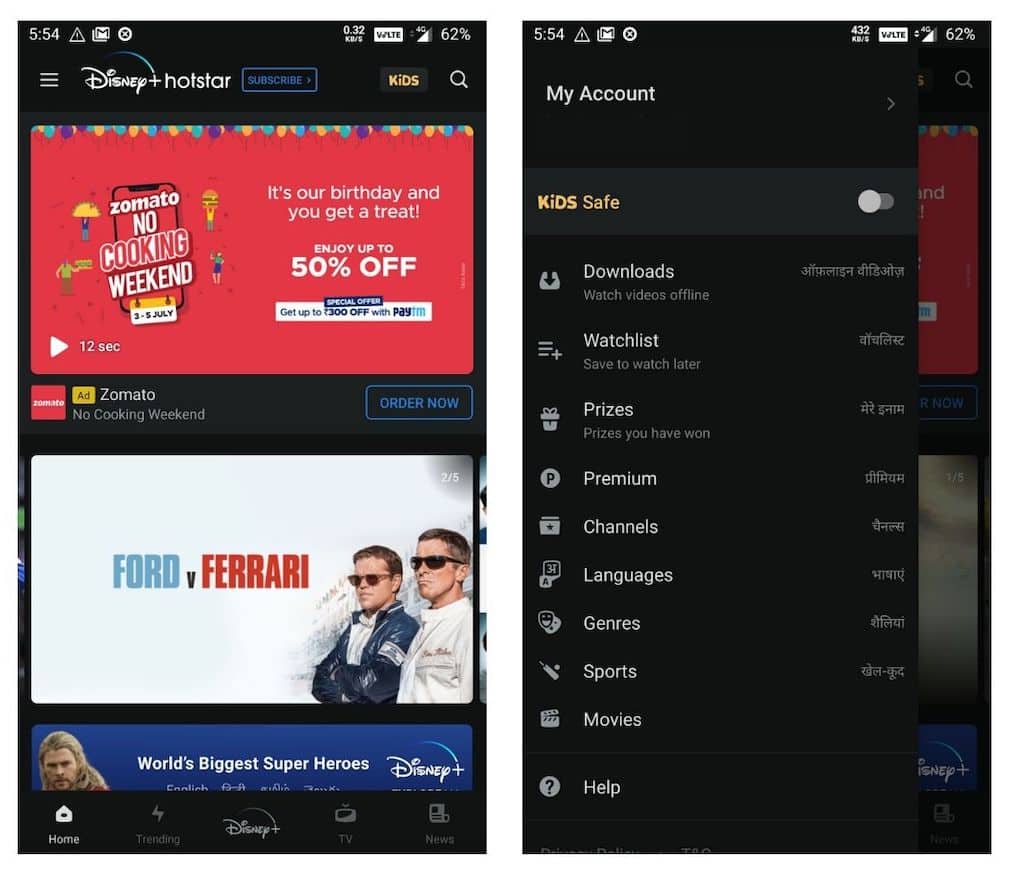Here is your requested detailed caption for the image:

---

The image consists of two screenshots taken from a smartphone. 

**First Screenshot:**
- **Timestamp and Battery:** The time displayed is 5:54 PM, with 62% battery remaining.
- **App Interface:** The interface shows the Disney+ Hotstar application.
  - A prominent blue button labeled "Subscribe" is visible.
  - Next to it, there are tabs named "Kids" and "Search."
- **Advertisement Box:** A distinct red box featuring promotional content from Zomato:
  - The top line announces "Zomato" in a stylized 'Z' font.
  - The text promotes a "No Cooking Weekend" from 2nd to 5th July.
  - Below, it mentions, "It's our birthday and you get a treat. Enjoy up to 50% off. Get up to $300 off with pay in."
  - Towards the bottom, in a black box, it repeats "Zomato No Cooking" with "Zomato" in red.
  - Instructions to "Order Now" are highlighted in a blue box.
- **Additional Promotions:**
  - An advertisement for the movie "Ford vs. Ferrari."
  - Another line promoting "The World's Biggest Superheroes" on Disney+.
  - An image of a man, likely related to the superheroes promotion.

**Second Screenshot:**
- **Disney+ Account Overview:**
  - The KidSafe button is activated.
  - Options listed include:
    - "Downloads (watch video offline)" - currently inactive.
    - "Watchlist" - to save content for later viewing.
    - "Prizes you have won."
    - Access to "Premium" content.
    - Categories such as "Channels," "Languages," "Sports," and "Movies."
    - A "Help" section for user support.

---

This detailed description is intended to provide comprehensive insights into the content and layout of the screenshots.